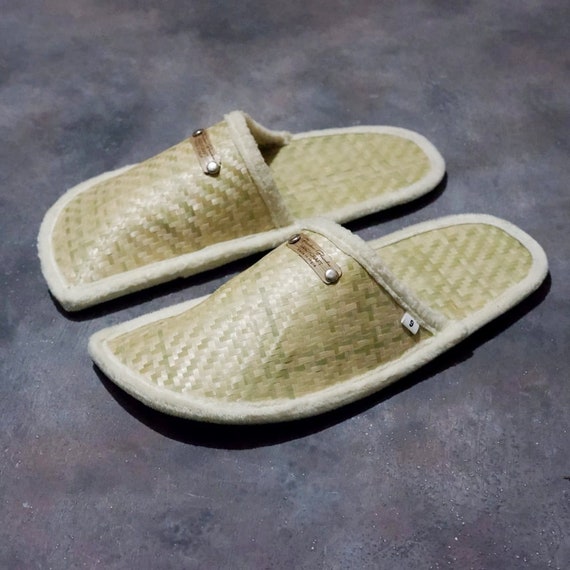The image captures a close-up of a unique pair of slippers made from woven straw or bamboo, displaying their intricate craftsmanship. The slippers are light brown, with interlaced patterns creating a fabric-like texture. They are adorned with a soft, fuzzy outer layer that encircles them, providing a gentle and plush appearance likely made from cotton. Each slipper bears a small rectangular label with two buttons on the top center portion, though the text is too small to read clearly. The slippers rest on a grey concrete floor, exhibiting a complex mix of bluish, reddish, and lighter grey shades. These hints of green within the woven material add an additional touch of color to the earthy tones predominantly seen in the image.